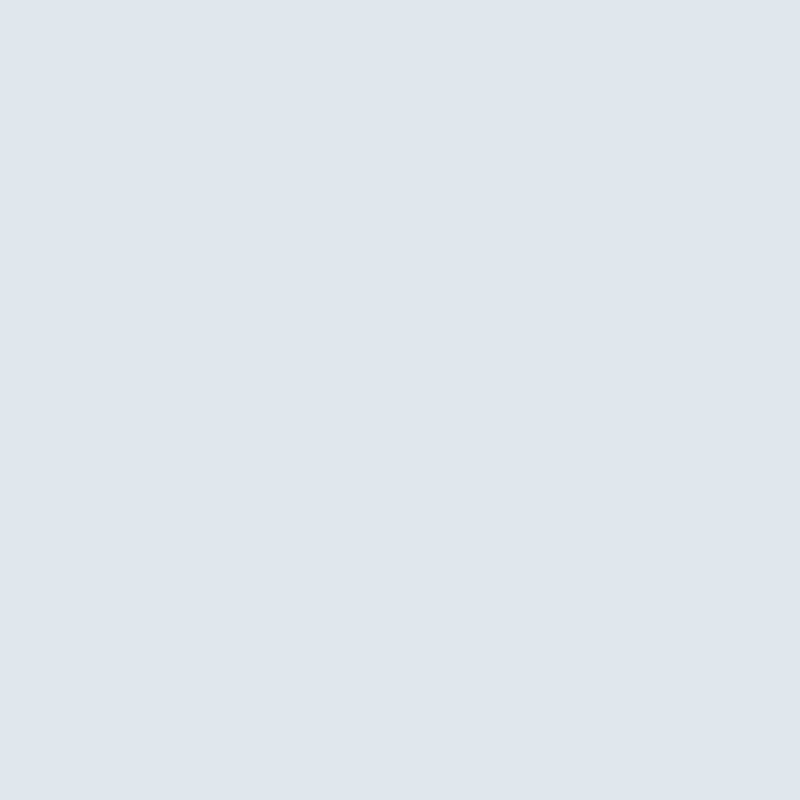The image presents a large, plain square of light blue color, occupying approximately six inches by six inches on the screen. The shade of blue bears a subtle hint of gray, distinguishing it from typical baby blue hues. The square is devoid of any text or pictures, and its soft, hazy tone evokes a calm, sky-like appearance. Because of its simplicity and lack of distinguishing features, it's challenging to ascertain whether it is a screenshot or a standalone graphic.